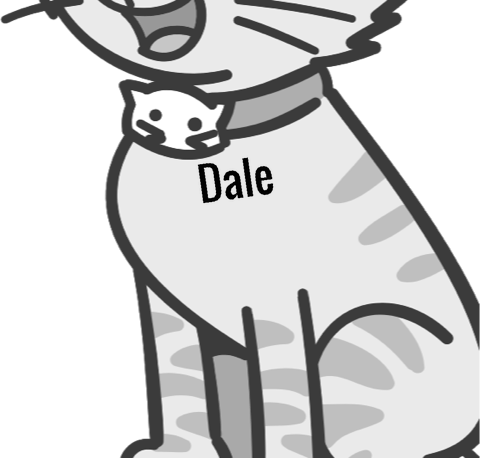In this detailed image, you're looking at a cartoon drawing of a light gray cat adorned with darker gray stripes running along its back, thighs, and front legs, each outlined in black for emphasis. The cat is seated upright, with its front legs resting on the ground. The visible portion of the drawing extends from just above the cat's open mouth, displaying its whiskers, down to about its paws. Around its neck, the cat wears a dark gray collar that features a white cat's face with black whiskers and eyes as a charm at the front. Just below the collar, the name "Dale" is prominently displayed in bold black letters, adding a personalized touch to this charming clipart.